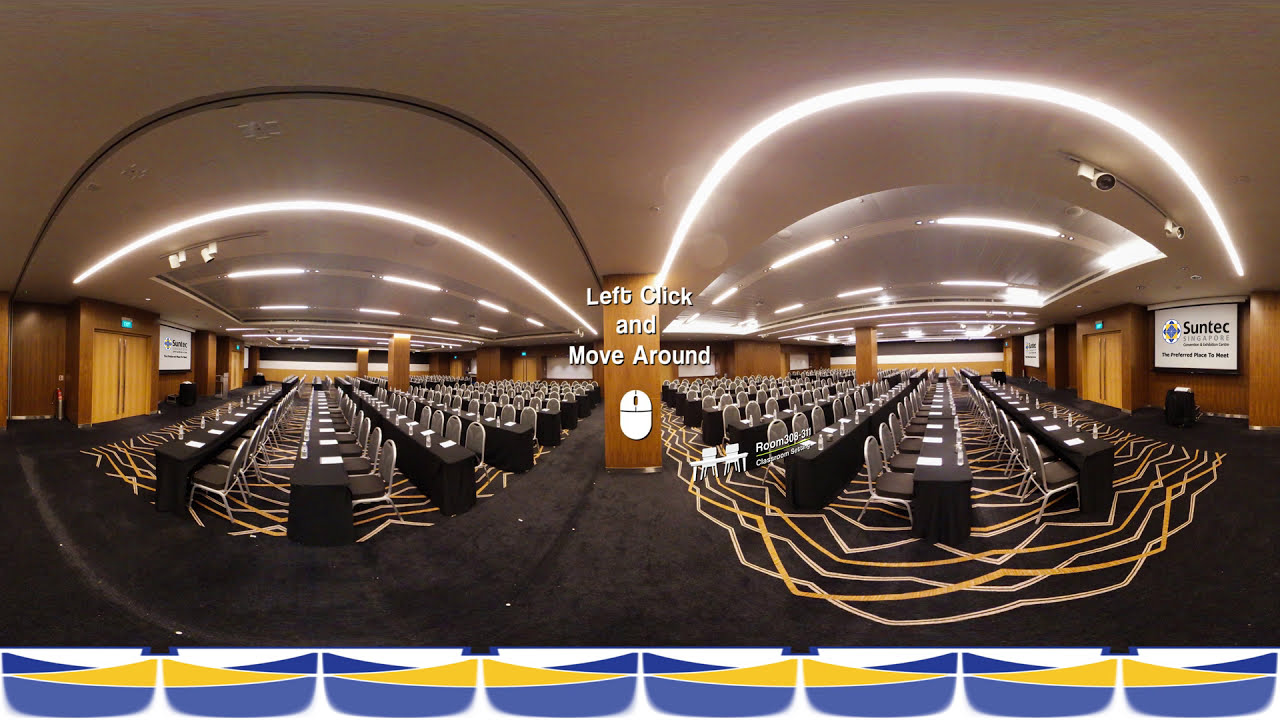This detailed photograph captures a spacious, conference-style auditorium with numerous silver and black chairs arranged in rows in front of black desks. Each desk is equipped with white notepads, bottles of water, and pens, ready for attendees. The room's design features a notable symmetry, with both the leftmost and rightmost walls made of a brown wood finish and featuring double doors with silver handles. 

The ceiling is white and adorned with rows of track lights stretching from the front to the back of the room, ensuring even illumination. Front and back projections display the word "SunTech" in black letters against a white background, accompanied by a blue, yellow, and white logo, indicating that this is likely a company event or meeting. An additional distinctive touch to the room's aesthetics is the carpet, which is gray with white and gold designs. The image appears slightly curved, suggesting it might be a capture from a VR environment, which would explain the unique visual perspective.

Overall, this setup indicates a well-organized space prepared for a formal gathering of potentially several hundred attendees, likely for training or a companywide conference focused on SunTech.